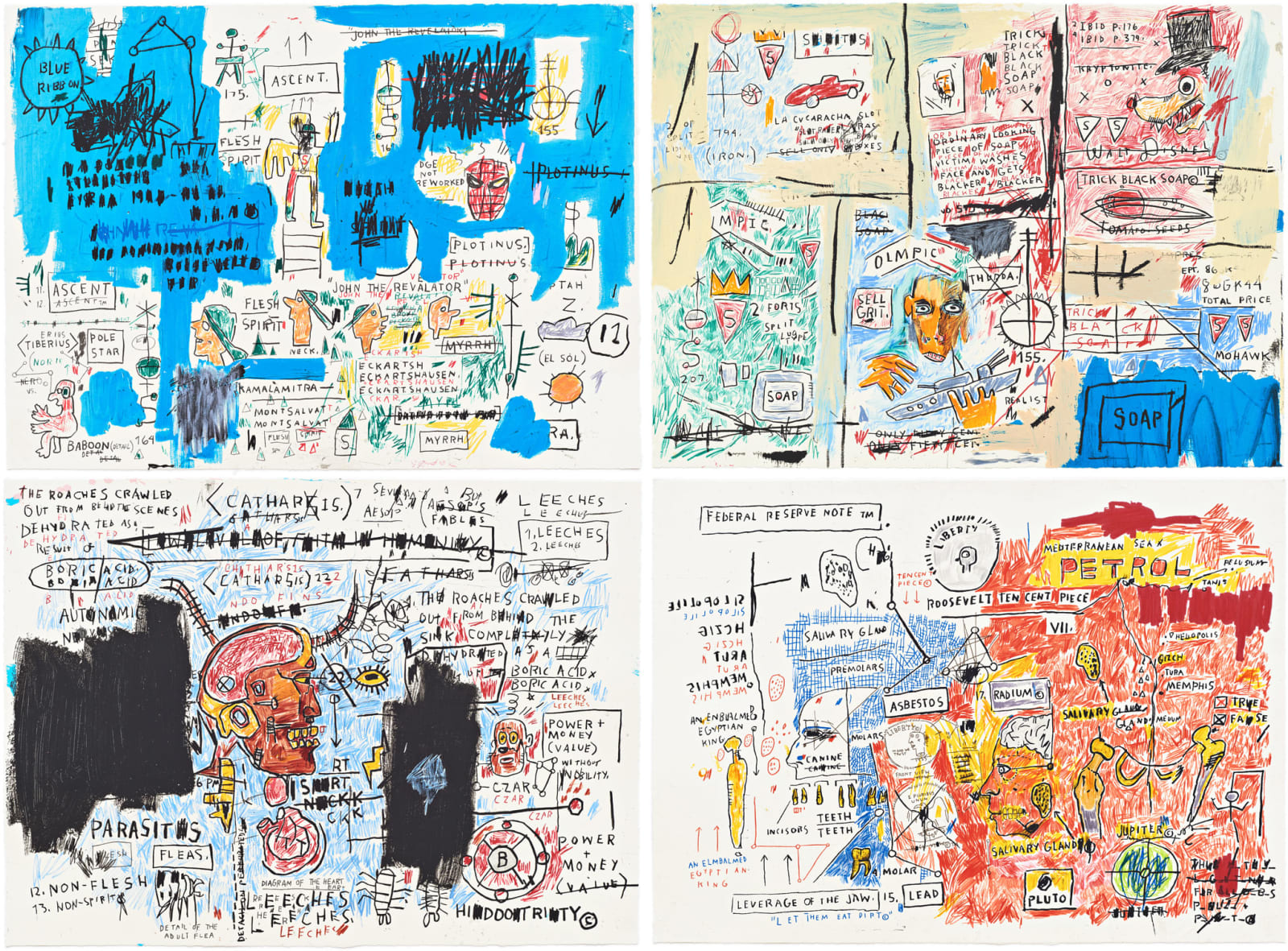Here, you have a collection of four chaotic and colorful drawings, each occupying a panel on what appears to be a poster board. The upper left panel is dominated by blue hues and features a splotchy background with various faces, including a Spider-Man mask, accompanied by the words "Ascent" and "Polestar." A sun and a blue ribbon are also tucked into the corner of this collage-like scene. The upper right panel showcases a man holding what looks like a tank or battleship, a blue square labeled "soap" above the word "Mohawk," and an ominous dog with fangs wearing a top hat, all set against a vibrant yellow background. The bottom left panel is densely packed with chaotic scribbles and random text like "parasites," "non-flesh," "non-spirit," "fleas," and "leeches." At its core is a detailed drawing of a head with an exposed brain and a heart outside the body. Lastly, the bottom right panel predominantly features red tones and includes the words "Federal Reserve note," "petrol," and "asbestos." Drawings of teeth, an explosion with flames, and planetary names like "Jupiter" and "Pluto" can also be seen. Overall, these drawings appear disordered, with childlike scribbles and a wide array of unsettling imagery and text running throughout.